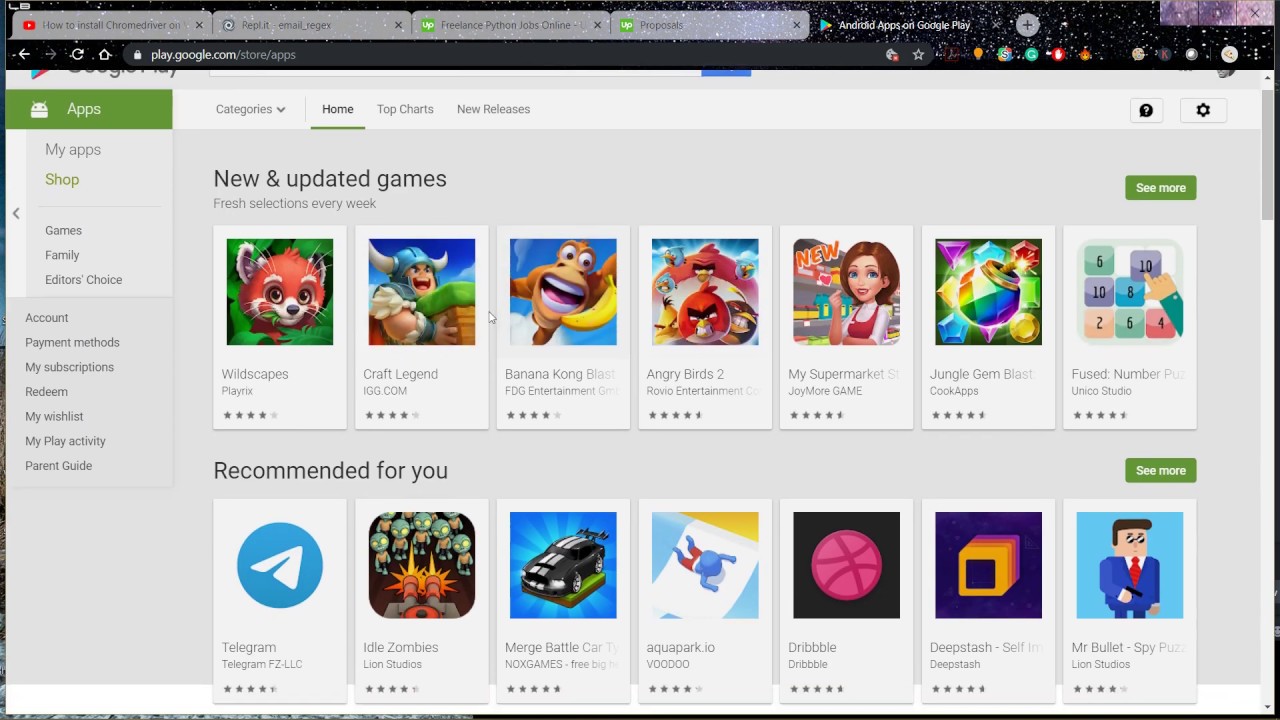This desktop screenshot captures the Google Play store, as viewed through a dark mode-enabled browser on a computer screen. The browser window showcases four tabs, though only one is clearly visible, with unreadable titles on the remaining tabs. The browser interface is designed with gray tabs and a striking black, star-field effect running along the right edge.

The Google Play store’s main content is the focus, set against a light gray background. On the left, a sidebar is prominently displayed featuring a green rectangle at the top, emblazoned with "Apps" in white text beside the white Google Android icon. Below that, the sidebar lists several categories in gray text: My Apps, Shop, Games, Family, Editor's Choice, Account, Payment Methods, My Subscription, Redeem, My Wishlist, My Play Activity, and Parent Guide.

The primary section of the store reveals two rows of game and app screenshots. The first row, headlined under "New and Updated Games," includes titles such as "Wildscapes," "Craft Legend," and "Angry Birds 2," identifiable by the well-known Angry Birds imagery. The second row, labeled "Recommended for You," starts with the Telegram app, identifiable by its distinct logo—a sky blue circle with a white paper airplane icon. Each row comprises approximately seven items, heralding a diverse array of recommended and updated games and apps.